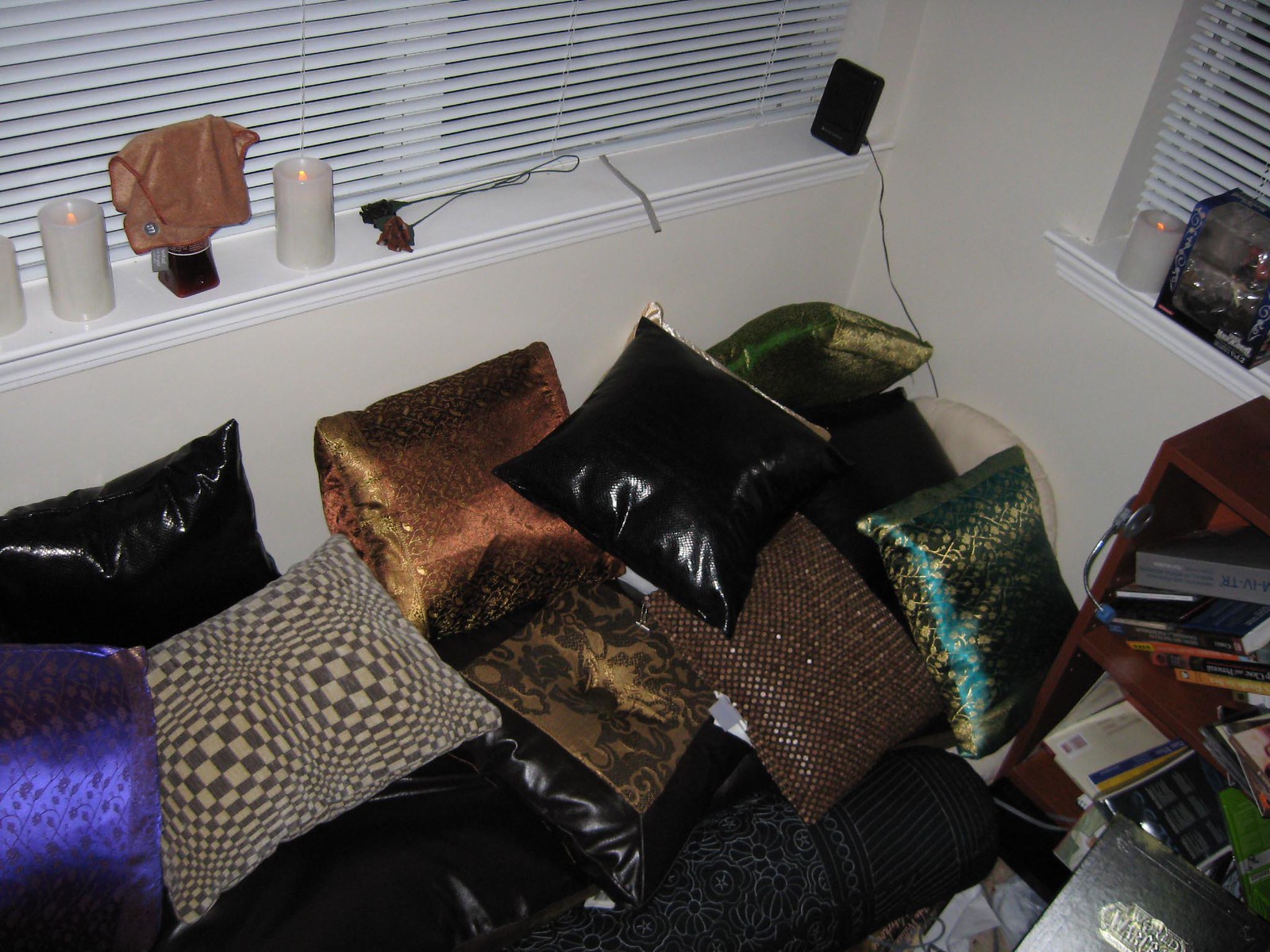This landscape-format color photograph captures a cluttered corner of either a living room or a bedroom, dominated by a large, eclectic pile of decorative cushions. The square pillows, all around 13 inches, vary dramatically in texture, color, and design. Among them are shiny black pillows resembling leather, blue satin ones with hints of yellow, green satin pillows, and others featuring intricate geometric patterns, including a checkerboard optical illusion with white and black. There's also a brown cushion embellished with sequins or small rhinestones and a tealish-green cushion with gold etching. The cushions, some dingy from use, are strewn across what might be a couch or bed with a black bedspread. This chaotic arrangement extends from the lower left of the frame up to the right corner.

The backdrop includes two white-painted windowsills adorned with small electric candles, some possibly lit, and the windows are fitted with closed white mini blinds. A phone can be seen charging on one sill. To the lower right stands a bookcase, filled haphazardly with books and other items. The walls are painted white, contributing to the relatively sparse decor outside the riot of colors and textures from the cushions.